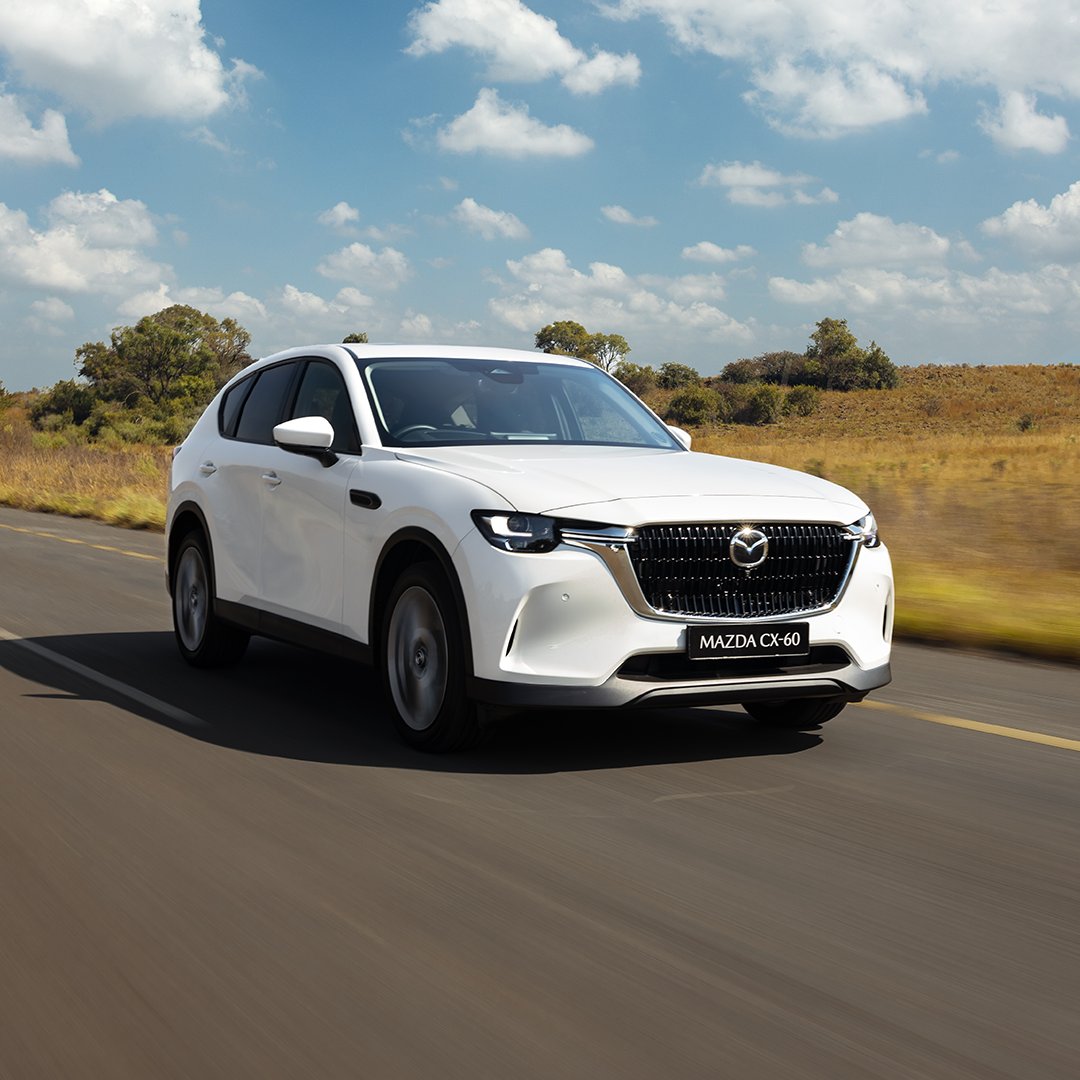The photograph captures an immaculately clean, white Mazda CX-60 SUV driving at a fair pace on a smooth road. The car, featuring regular silver wheels with its model name clearly displayed on the front number plate, is moving toward the camera. The movement is evidenced by the blurred hubcaps and slight motion blur in the surrounding landscape. The backdrop reveals a natural scene with shades of brown and yellow grass, a few green trees, and some bushes, indicative of scrubland or a deserty area. Above, the sky is a vibrant blue dotted with numerous white, puffy clouds, suggesting a beautiful summer day. The composition and quality of the image resemble those typically seen in manufacturer press releases or on official car dealership websites, emphasizing a polished, professional style.